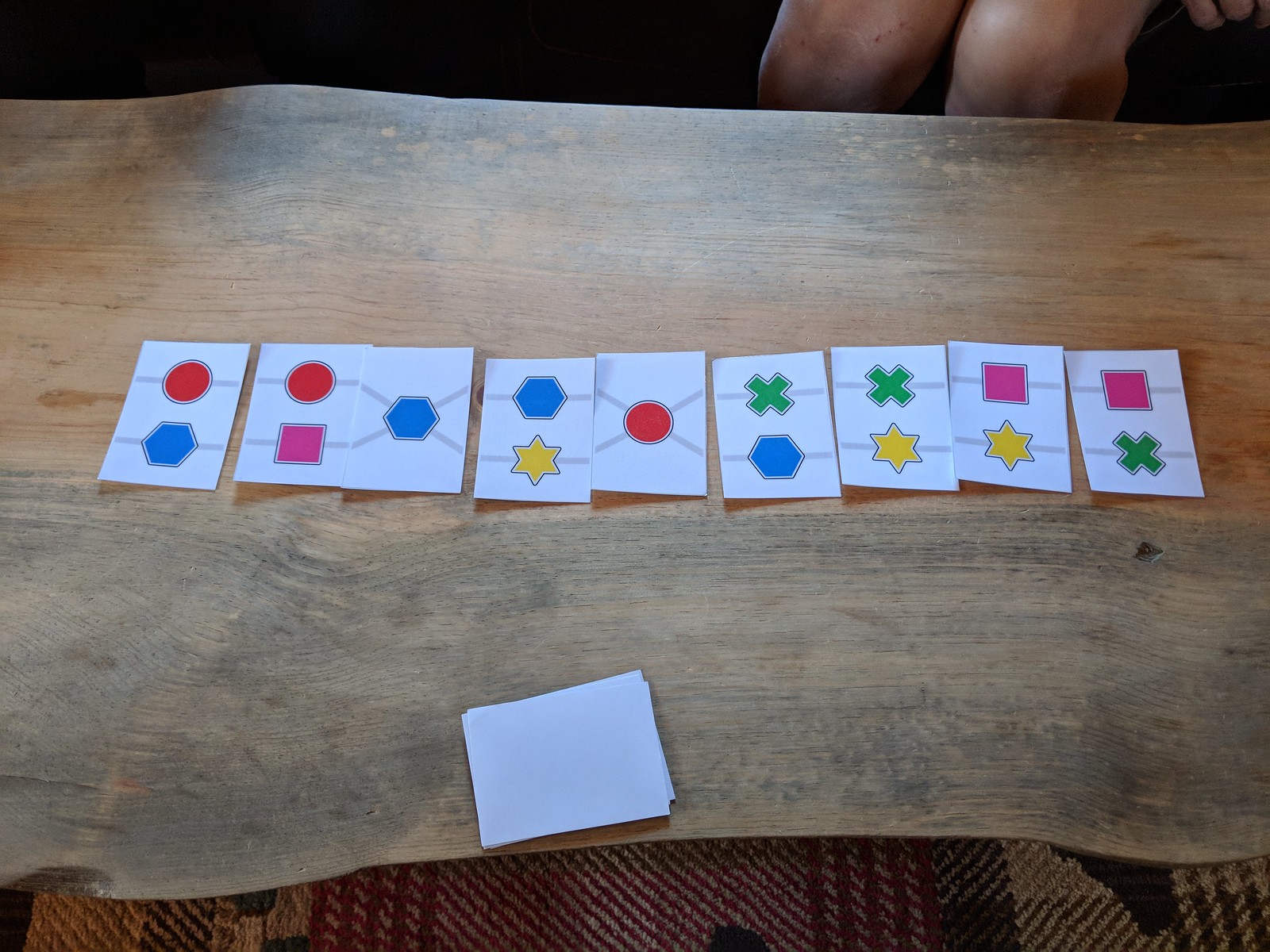A rustic wooden coffee table, crafted from a lengthwise-cut log and carefully sanded, sits in the center of this cozy scene. At the table's top-right corner, a glimpse of two knees and a few knuckles hints at a person seated across from the photographer. Below the table, a mysterious black shape, possibly a sock or part of the rug, adds an element of curiosity. The rug itself is an intricate tapestry of red, white, black, and creamy colored stripes. 

Upon the table, ten cards are arranged in a meticulous line, suggesting a game in progress. Below this linear formation, a small stack of cards lies face down, ready for the next move. The cards are adorned with lines and symbols that appear to need alignment—circles matching circles, lines connecting lines, forming a pattern that probably dictates the rules of the game. This thoughtful arrangement and the warm, homey setting suggest a moment of quiet engagement and enjoyment.